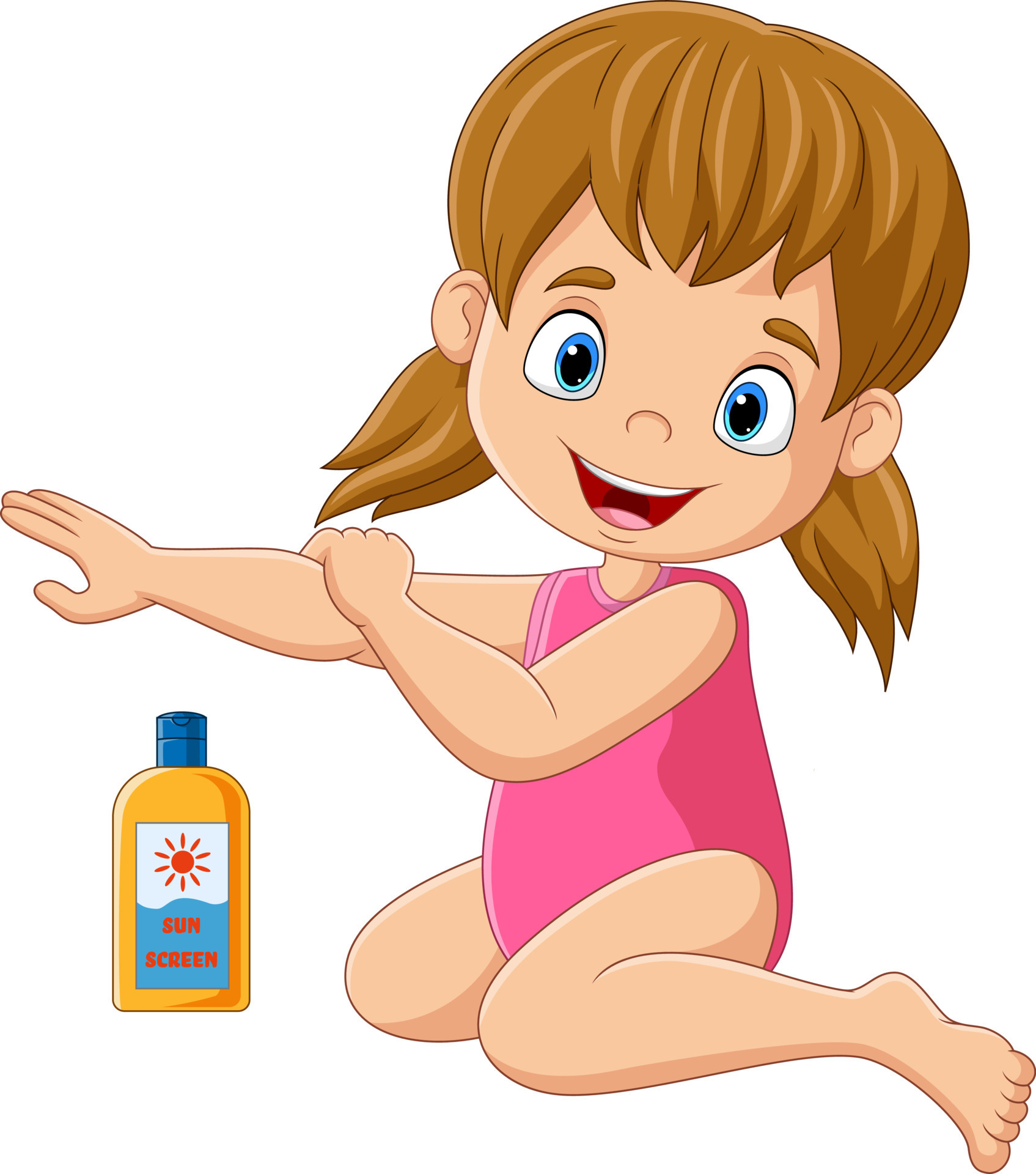This is a detailed cartoon drawing of a young girl, likely around three or four years old, who is smiling warmly at the viewer. She has large, expressive blue eyes, brown eyebrows, and medium-length golden brown hair that falls around her shoulders. The girl's skin is cream-colored, and she is dressed in a one-piece pink swimsuit. In the drawing, she is depicted sitting down and applying sunscreen to her right arm with her left hand. 

To her left, there is a prominently placed yellow bottle of sunscreen with a blue cap. The bottle has a label with the word "sunscreen" written in red letters. The label also features an illustration of the sun above a blue background that resembles the ocean, and the bottle appears to contain an orange liquid. The entire scene is set against a plain white background. The detailed elements in the image highlight the importance of sun protection, portraying the girl as knowledgeable and diligent in applying sunscreen to avoid sunburn.